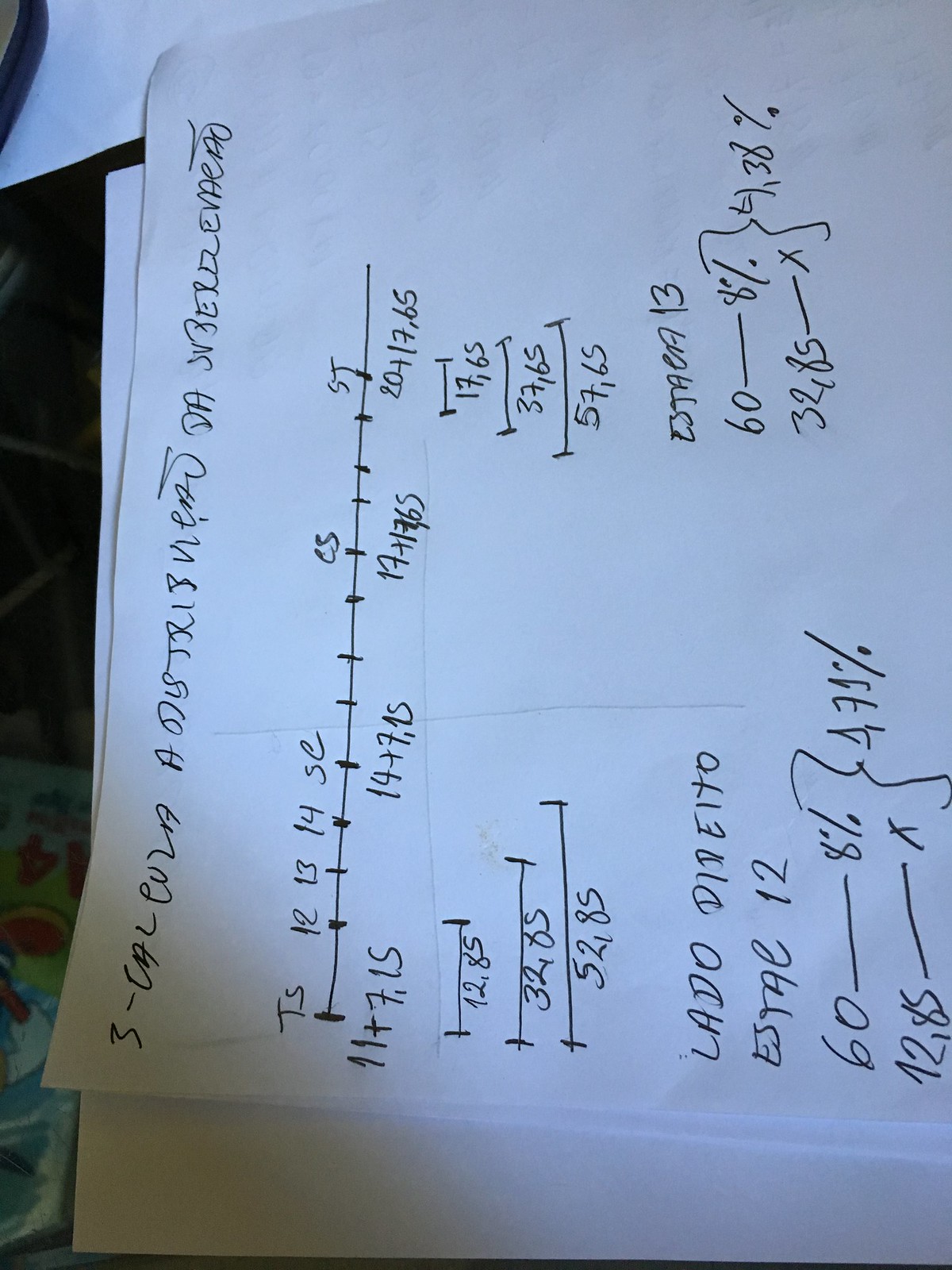The photograph depicts a handwritten page filled with various notes, diagrams, and calculations. The language of the notes is non-English, suggesting the content might be specific to a particular region or discipline. Central to the page is a long line divided into multiple segments, each annotated with distinct labels such as "TS," "12," "13," "14," "SC," "CS," and "ST." Additionally, there are lines with dashes at both ends, bearing numerical inscriptions beneath them like "12,085," "12.85," "32.05," and "52.85," indicating possible measurements or calculations.

Towards the bottom of the page, a series of equations are visible, characterized by the use of parentheses, percentage signs, and placeholders denoted by Xs. These equations appear to be part of a larger mathematical or scientific problem. The entire content is meticulously handwritten in a dark pen, adding a personal touch to the detailed and complex information conveyed on this piece of paper.